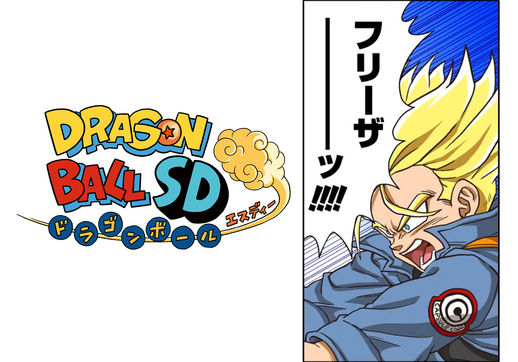The image is divided into two distinct sections. On the left, there is a digital print featuring the text "Dragon Ball SD." The word "Dragon" is displayed in yellow text with a blue outline, "Ball" in red text also with a blue outline, and "SD" in blue text bordered in black. Below this text, there are seven blue circles with intricate geometric designs inside them. Additionally, there's a yellowish-beige puff of smoke emanating to the right side of the text.

On the right side of the image, a tall rectangular section showcases a man with distinctive blonde hair that's spiked and has a blue tint at the top. He's dressed in a dark blue, almost gray, jacket with a patch on it. He appears to be holding something, potentially a steering wheel, and has his arms extended forward. The man’s expression is intense, with his mouth slightly open as if snarling, and his hair streams upward and to the right. The white background of this section features some black Asian text in the upper left corner.